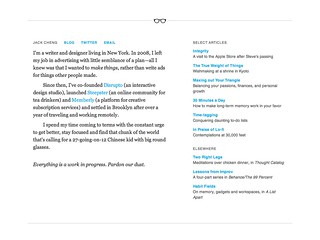In this blurry image, we can make out an excerpt from what appears to be a blog post. The text is extremely fine, necessitating zooming in to decipher the content. The first visible paragraph mentions someone named Jack, though the last name is unreadable. The text reads: "I'm a writer and designer living in New York. In 2006, I left my job in advertising because I wanted to make a significant change." The remainder of the paragraph is too small to read.

The layout of the image suggests that the left side features three paragraphs of the aforementioned blog post, though their content remains largely illegible. On the right, there appear to be additional articles, but their titles and details are also too tiny to discern. The image predominantly uses a monochromatic color scheme with black and white text, highlighted with some blue font elements.